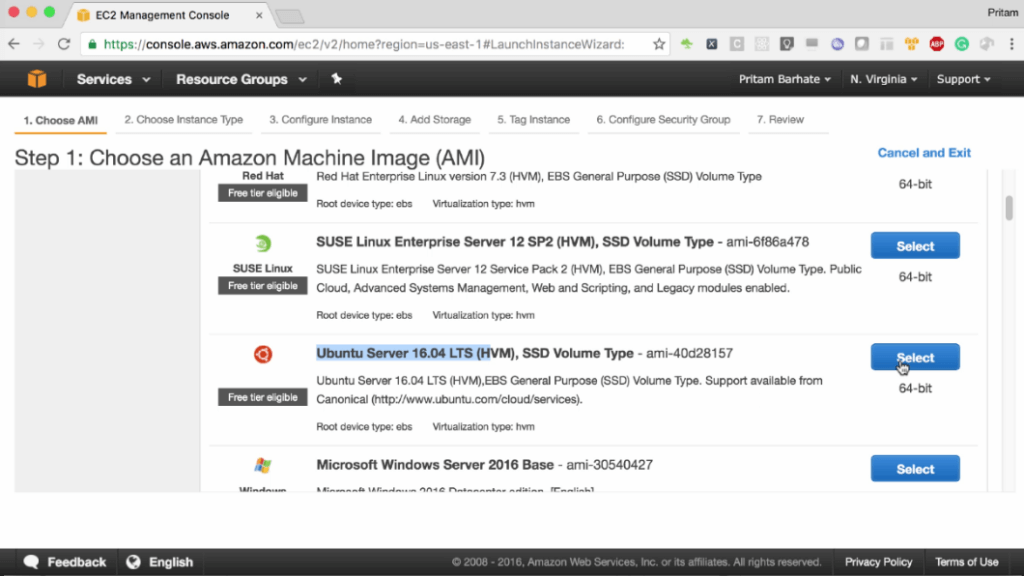The image captured from the website console.aws.amazon.com shows the EC2 Management Console in a web browser. In the top-left corner of the browser tab, there are three control circles: red, yellow, and green. Below the tab, the interface features a gray rectangle spanning the top section, with a black rectangle just underneath. 

The primary content area is predominantly white, bordered by a vertical gray rectangle on the far left side of the screen. At the bottom of the image, there's a black rectangle that includes links for Feedback, English language selection, Copyright, Privacy Policy, and Terms of Use.

Focusing on the main content, the heading indicates "Step 1: Choose an Amazon Machine Image (AMI)," listing several operating system options such as Red Hat Enterprise Linux, SUSE Linux Enterprise Server, Ubuntu Server, and Microsoft Windows Server 2016 Base. The option for Ubuntu Server is highlighted, and the cursor hovers over the "Select" button, which is displayed in blue.